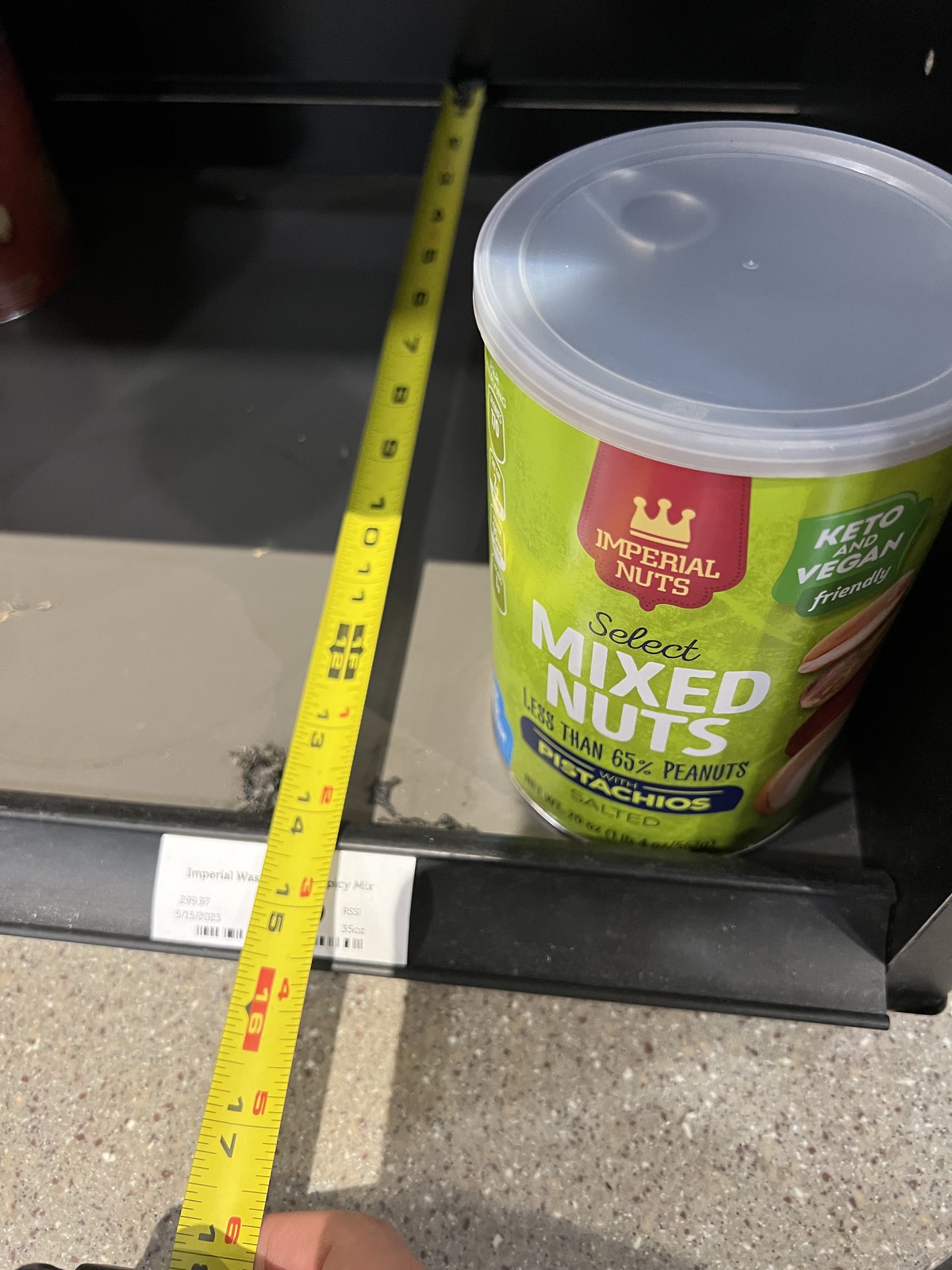The image features a central focal point of a yellow measuring tape encased in a pink container, stretched horizontally across a dark gray background. The tape is marked with black numbers. Next to the tape, there's a gray tray with an outer darker gray and an inner lighter gray finish. Inside the tray sits a green can labeled "mixed nuts" in white letters. The can has a plastic lid and a silver pull-top seal visible underneath. A small red sign on the side of the can reads "Imperial Nuts" and is adorned with a gold crown emblem. The entire arrangement rests on a surface that appears to be a speckled gray granite, adding a touch of texture to the composition.